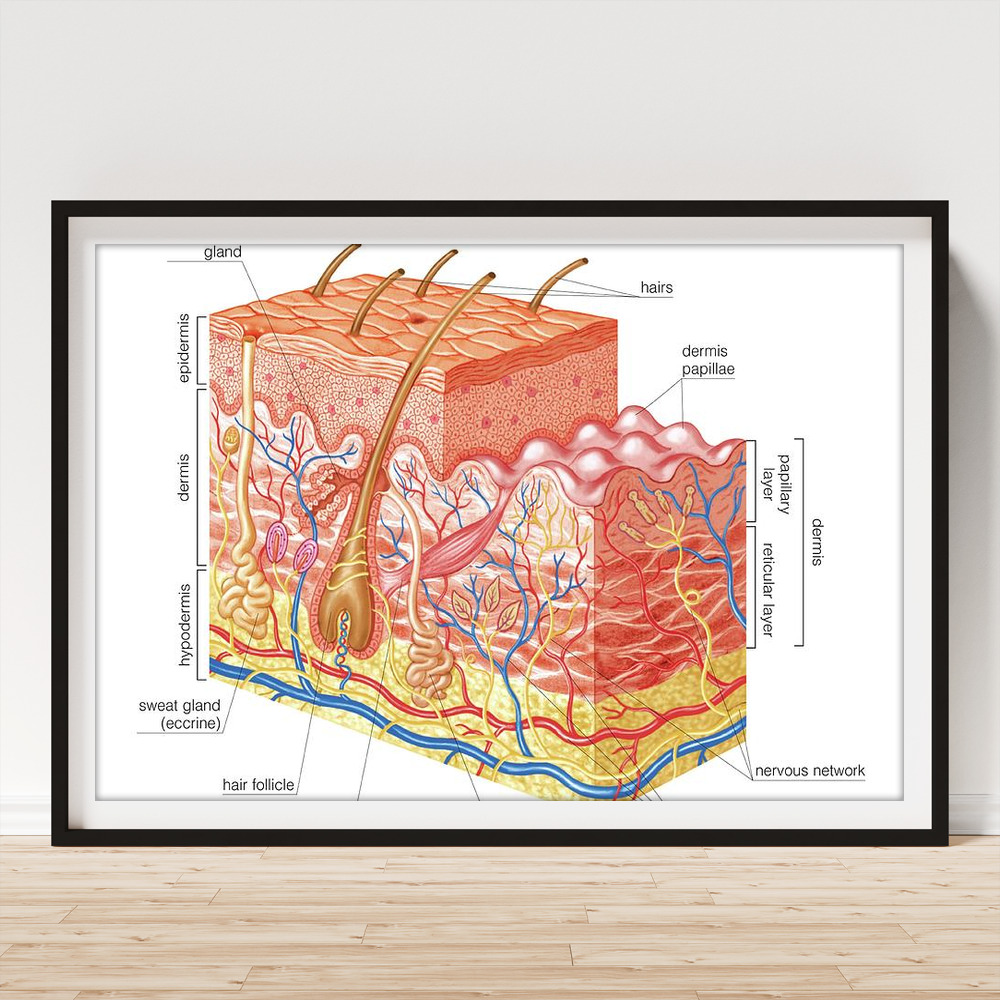This image displays a black-framed, white-matted, cartoony-style anatomical diagram of human skin, leaning against a plain white wall on a light-colored wooden floor. The wooden boards feature a grain pattern running diagonally from the lower left to the lower right. The diagram showcases an array of vivid colors, including pink, yellow, blue, and red, and details various cutaway anatomical parts labeled with text such as 'epidermis,' 'dermis,' 'hypodermis,' and 'sweat gland.' It highlights the nervous network, hair follicles, hair roots, blood vessels, and different layers of tissue, including the reticular layer and the papillary layer.